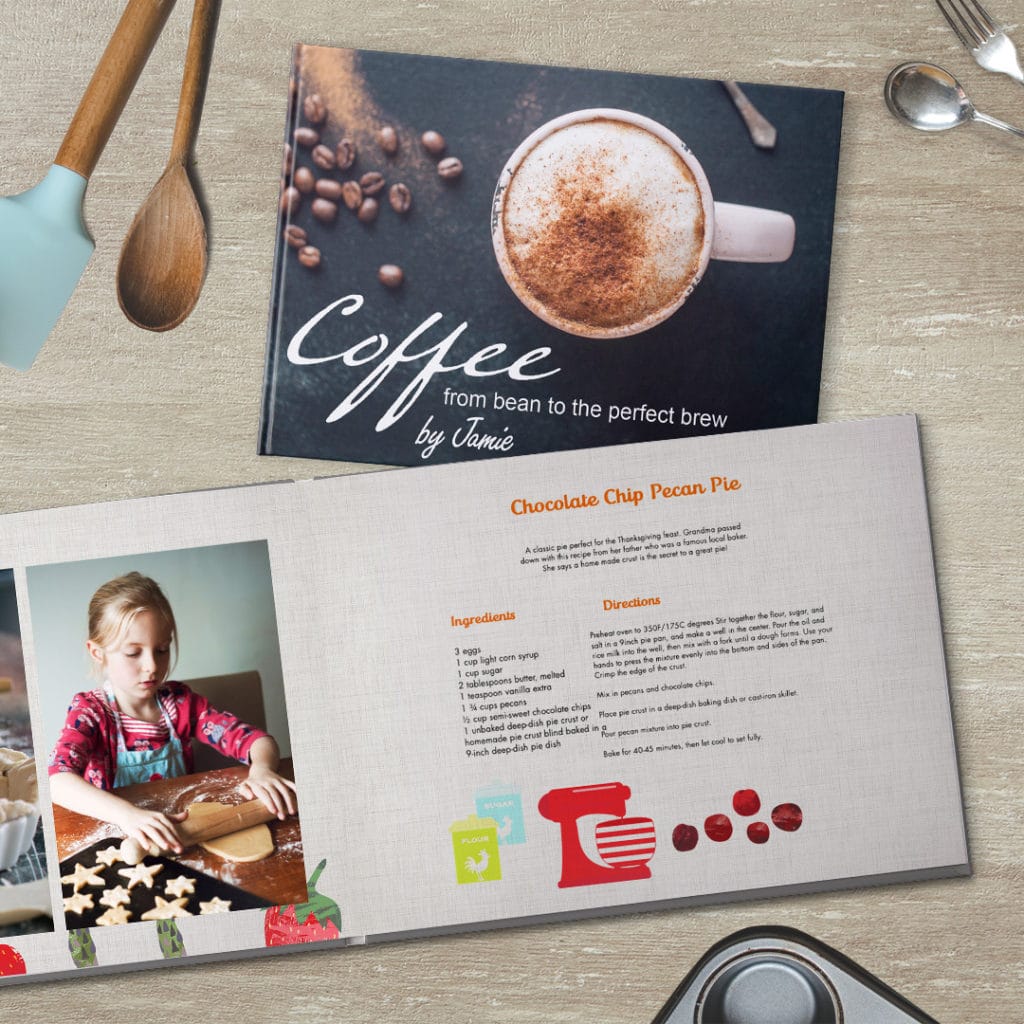On a gray wooden table, there are two books prominently featured. The top book has a black hardcover with a white cup of coffee pictured on it, showcasing a detailed top-down view that includes whipped cream and a sprinkle of nutmeg. Surrounding the cup are scattered coffee beans and a dusting of nutmeg on a black surface. The cover text reads "Coffee: From Bean to the Perfect Brew by Jamie," with the author's surname partially obscured. Below, there's an open book displaying a recipe for "Chocolate Chip Pecan Pie." On the left page, there's a vivid illustration of a young girl, around nine years old, with blonde hair. She is clothed in a blue apron over a reddish shirt and is using a wooden roller to flatten star-shaped dough on a black tray. The right page of the book provides a detailed recipe, complete with ingredients like eggs, light corn syrup, sugar, and butter, accompanied by instructions on how to prepare the pie. Adjacent to the books on the table, various kitchen utensils, including a fork, a spoon, and other wooden tools, are scattered. The scene is meticulously arranged to convey a cozy and inviting baking atmosphere.